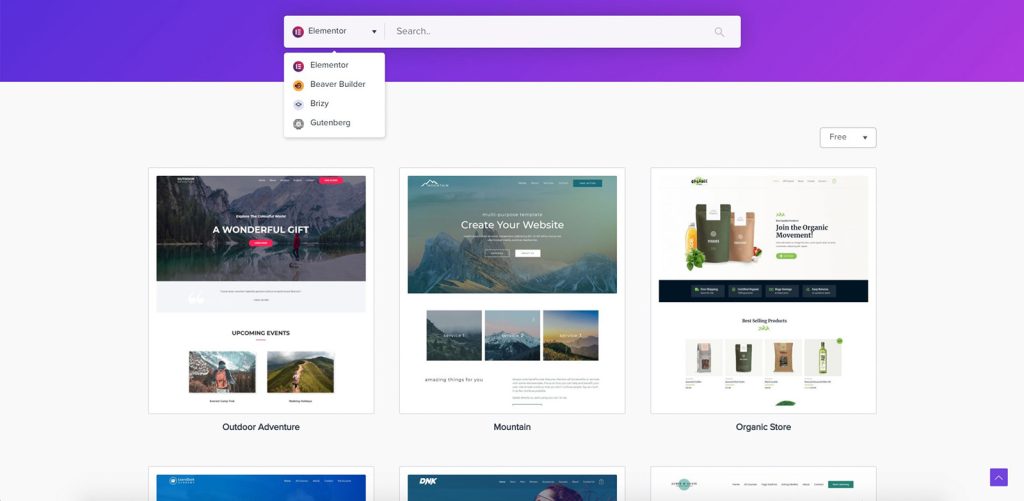The image depicts a screenshot of a website interface. At the top of the screen, there is a gradient purple header containing a central search bar with a drop-down menu on its left side, offering various options for the user. Below the header, the background shifts to white, showcasing different website format options. 

The first template, titled "Outdoor Adventure," is positioned on the far left. It features nature-themed images, including majestic mountains, accompanied by the text "A Wonderful Gift." 

The second template is labeled "Mountain." It has an image of towering mountains at the top with the text "Create Your Website" prominently displayed.

The third template, named "Organic Store," displays images suggestive of reusable bags and contains text that is unfortunately too small to decipher.

In the bottom right corner of the screenshot, there is a purple square with a white arrow pointing upwards, likely indicating an interactive element or button.